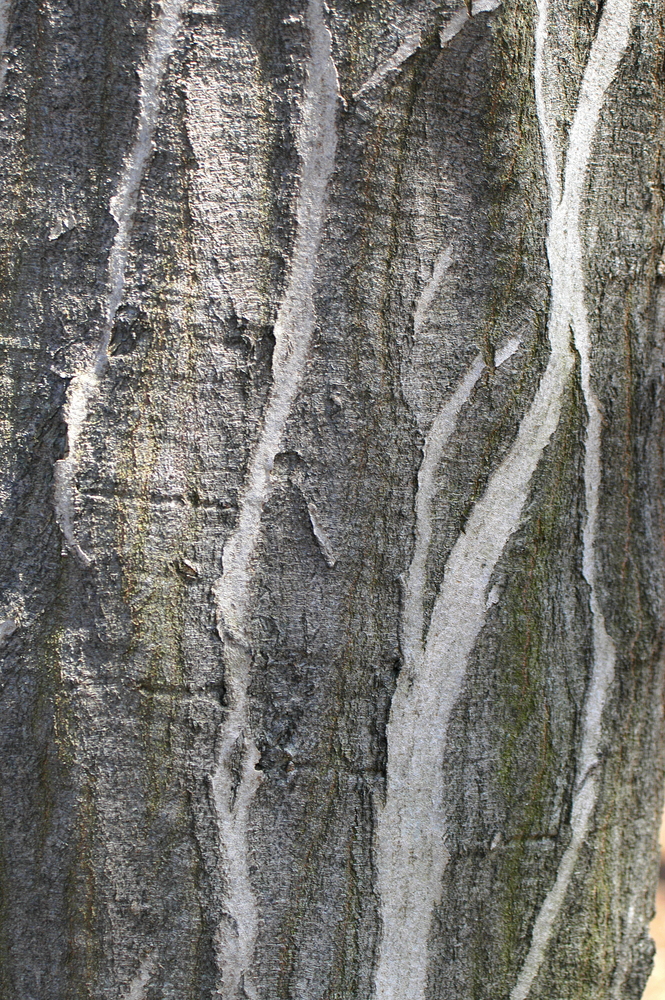The image is a detailed close-up of the bark of a European hornbeam (Carpinus betulus), capturing its distinctive and unique texture. The bark features a smooth background, contrasting sharply with vertical whitish-gray stripes that resemble ribbons or bands, giving it a striped appearance similar to rock. These vertical stripes run from the top to the bottom of the image, highlighted against the deeper gray, rough, and sandpaper-like surface beneath. The bark also displays additional colors; brownish-red streaks and portions of green moss suggest a natural aged patina. The photograph, bathed in sunlight, creates reflections that brighten certain parts of the bark, enhancing the visual texture and depth. On the far right edge of the image, a sliver of sunlight peeks through, illuminating a small section of the ground. This highly detailed close-up emphasizes the aging and complex pattern of the tree's bark, complete with cracks, divots, and mossy growths, making it appear both ancient and textured.